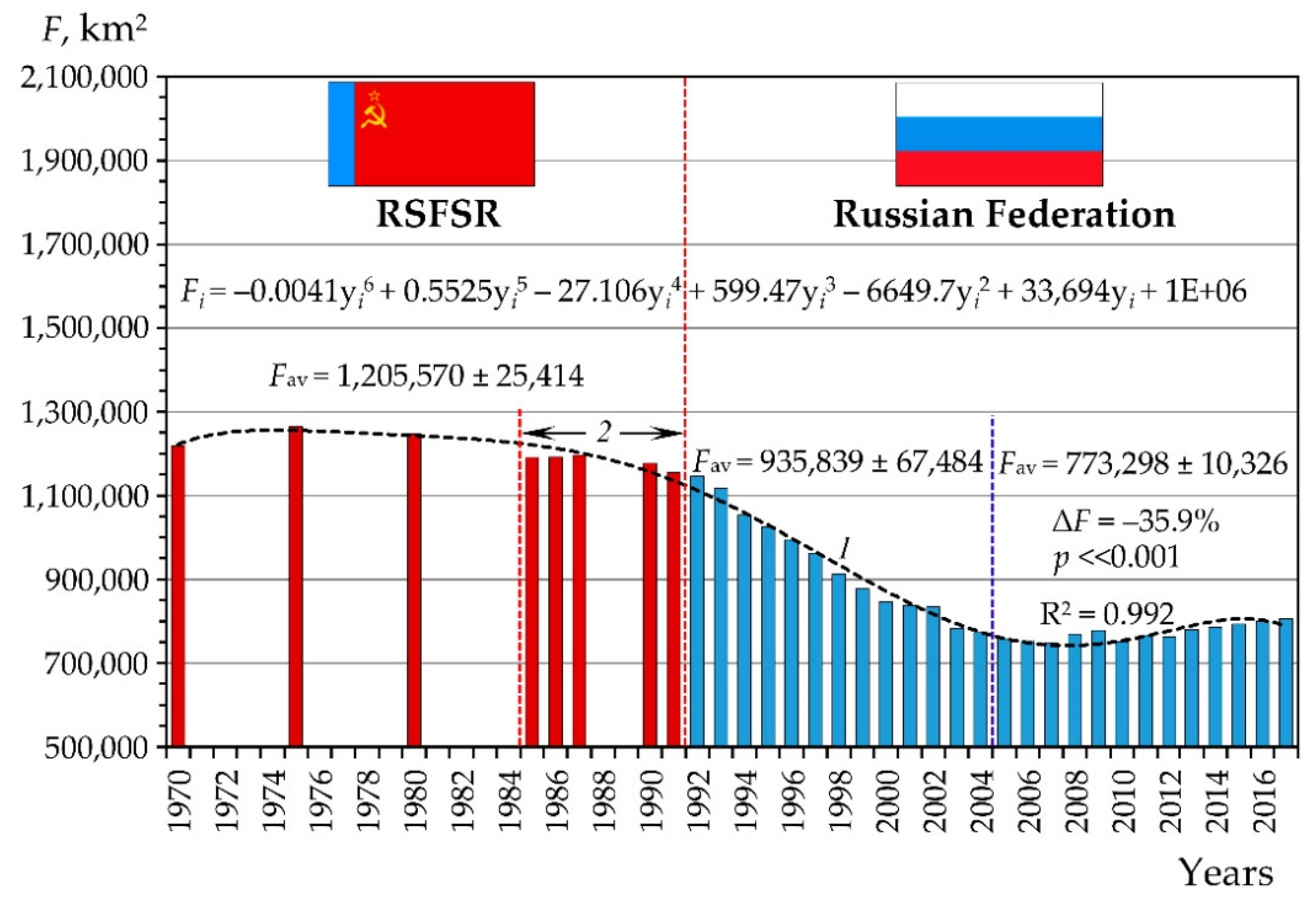The image depicts a detailed bar graph comparing the RSFSR (using the flag of the Soviet Union, red with the sickle and hammer in gold) and the Russian Federation (using the flag of Russia, with white, blue, and red bars). The x-axis spans from 1970 to 2016, marked at two-year increments, while the y-axis measures in square kilometers (F, km²) ranging from 500,000 to 2.1 million. The graph incorporates various complex mathematical formulas and calculations, shown to the right. The left half, representing the RSFSR, is characterized by red bars, whereas the right half, representing the Russian Federation, features more stable and consistent blue bars. Notably, there are gaps in the RSFSR data indicating missing values for certain years.